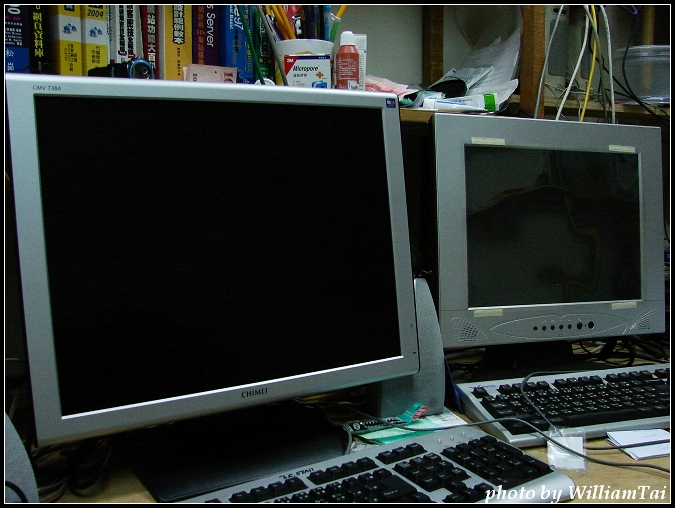In this detailed image of an office or workplace, two older desktop computers with side-by-side monitors are prominently featured. Both monitors have a gray exterior with the left one slightly larger, branded CHIMEI, and the right monitor without a visible brand. The screens are turned off, showing a black color. Below these monitors are two identical QWERTY keyboards with black raised keys set in a gray, stainless steel-like body. A notable small gray speaker is positioned between the two monitors. 

Above the setup, a shelf is filled with various IT-related books and miscellaneous items—such as a cup holding pencils and other utensils, a wristwatch, a clear container, and tubes that might be first-aid cream—suggestive of an IT office environment. More clutter includes some money scattered on the shelf. Tangled wires of gray, yellow, white, and black hang down from the setup, adding to the desk’s slightly messy appearance. Additionally, there are small papers and notepads placed next to the keyboards, with a specific white notepad in front of the keyboard on the right side. The entire setup sits on an older desk, and the bottom of the photo credits William Tai as the photographer.